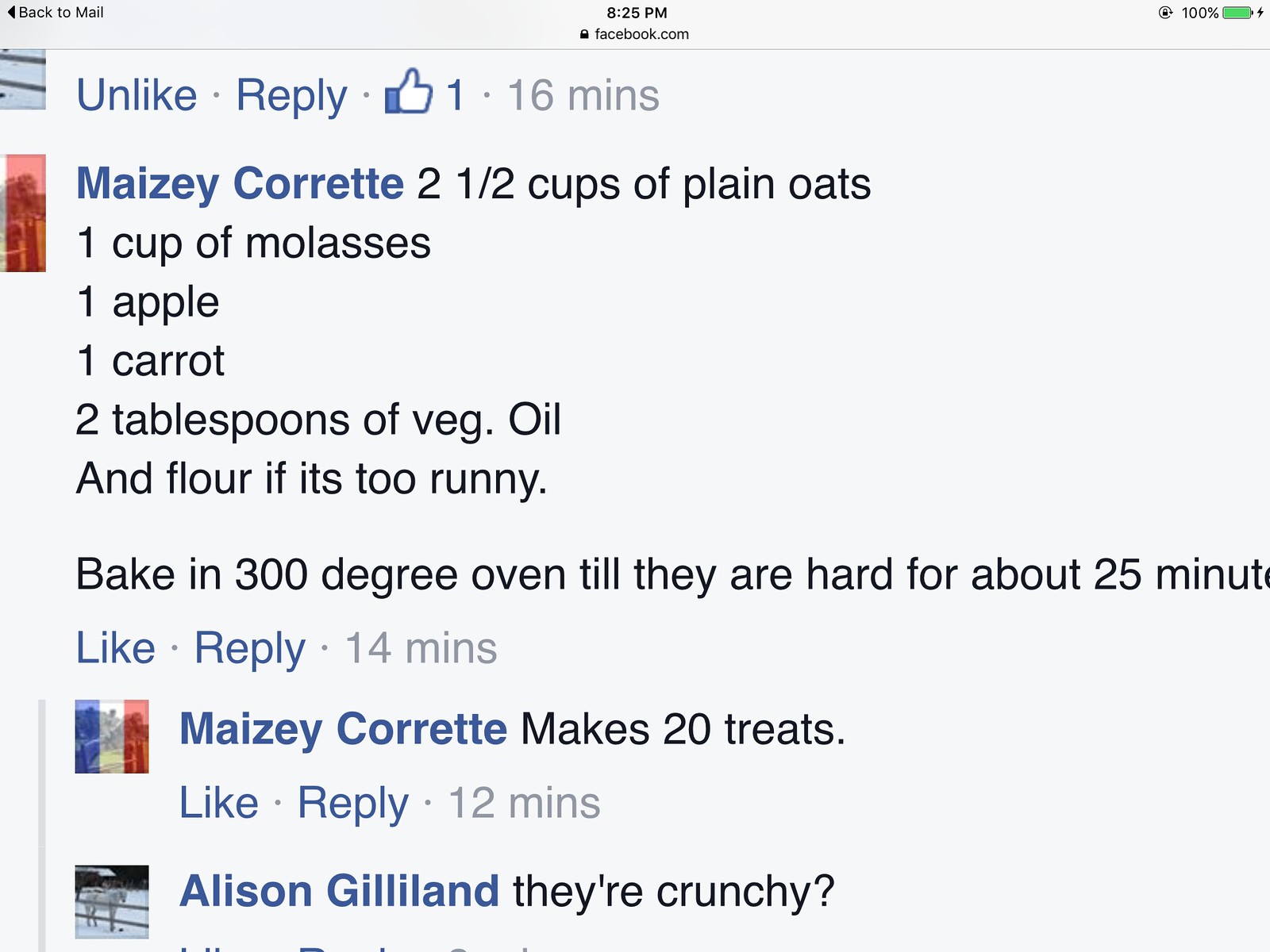The image is a screenshot of a recipe posted on Facebook by Maisie Koret. Her profile picture includes an icon showing the French flag superimposed over a historical photo. The recipe calls for 2.5 cups of plain oats, 1 cup of molasses, 1 apple, 1 carrot, and 2 tablespoons of vegetable oil, with a note to add flour if the mixture is too runny. It instructs to bake the mixture in a 300-degree oven for about 25 minutes until they are hard, yielding 20 treats. The entire screen is tinted a very pale blue. Below the recipe, a user named Allison Gilliland, whose profile picture features a white horse behind a fence, comments, asking if the treats are crunchy. The post has no likes but does have a couple of replies, with timestamps indicating recent activity.